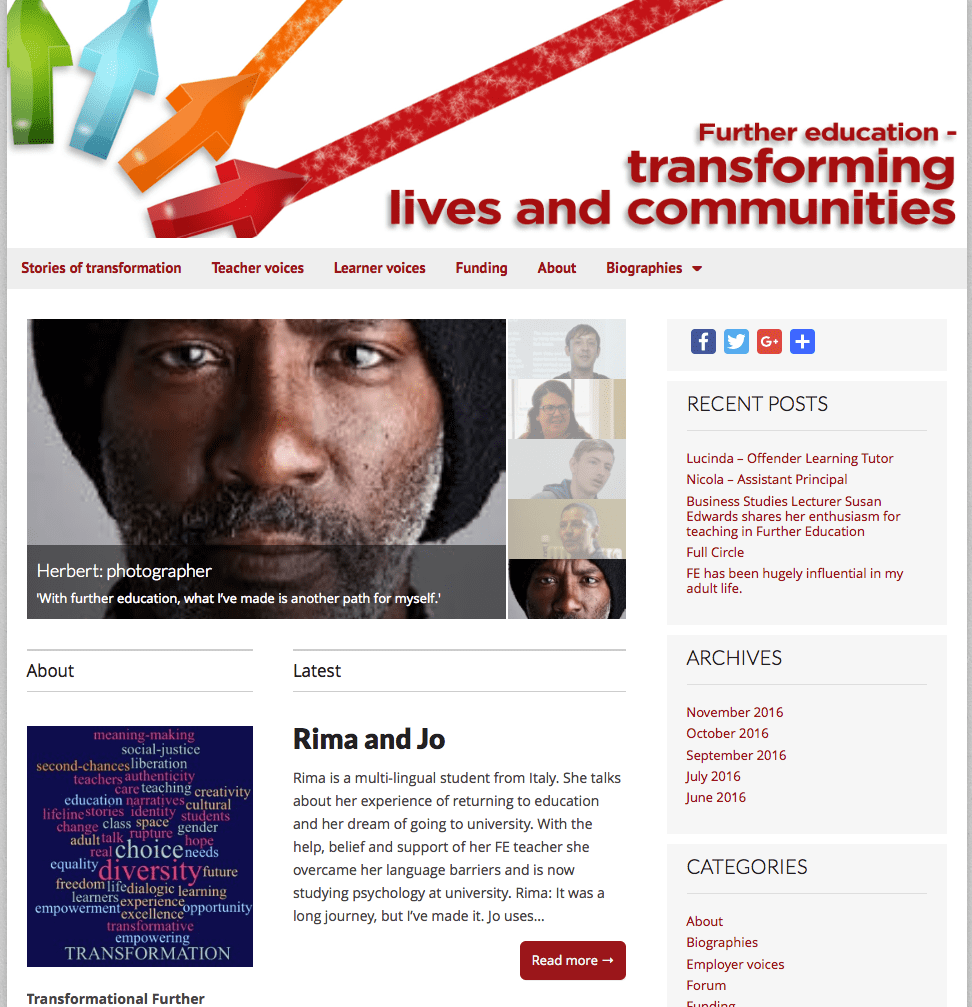The image showcases a screenshot from an educational website, though its exact name isn't identifiable due to the absence of a clear logo or website title. The top of the page features a motivational text stating, "Further education, transforming lives and communities." Below this header, the navigation menu offers several links including Stories of Transformation, Teacher Voices, Learner Voices, Funding, About, and Biographies.

Dropping down the page, there are numerous thumbnail images of individuals, likely educators or key figures involved in education. The right sidebar contains sections for Recent Posts, Archives, and Categories, providing structured navigation options. Toward the left-center of the page, distinct headings titled About and Latest are present. The highlighted content under the Latest heading includes a brief story titled "Rima and Joe," which appears to narrate the experiences of Rima, a multilingual student from Italy, detailing her journey and experiences in further education.